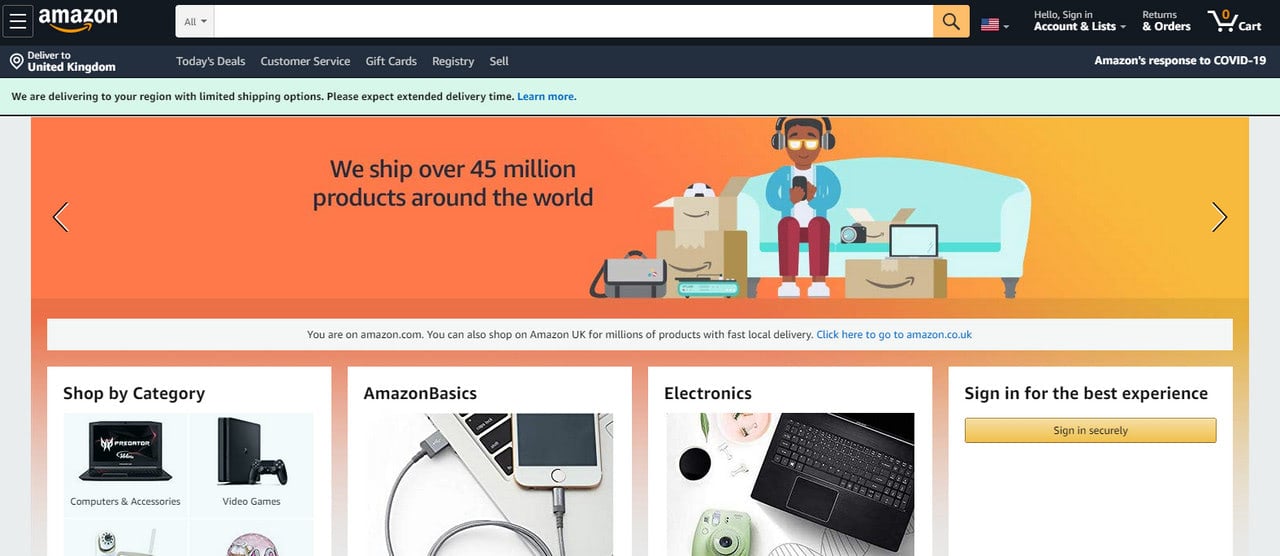The Amazon homepage presents a classic, albeit somewhat cluttered, appearance. Dominated by a large search bar at the top, the page is interspersed with numerous blue elements, creating a dense visual. Above the search bar, a prominent banner declares, "We ship over 45 million products around the world." This banner features a whimsical, computer-generated image of a Black man sitting on a blue sofa, wearing headphones and holding a TV remote, surrounded by Amazon boxes.

Directly below the banner, sections such as "Shop by Category," "Amazon Basics," and "Electronics" are highlighted, alongside a prompt encouraging users to sign in for the best experience. The cart icon is visible but remains empty as the user is not signed in. In the "Shop by Category" section, items like computers and accessories, video games, electronics, a digital camera, and a laptop are partially displayed.

Beneath the search bar, a message states, "Deliver to United Kingdom," noting, "We are delivering to your region with limited shipping options, please expect extended delivery time," accompanied by a "Learn More" link for further information. On the right side of the page, there's a link providing details on Amazon's response to COVID-19.